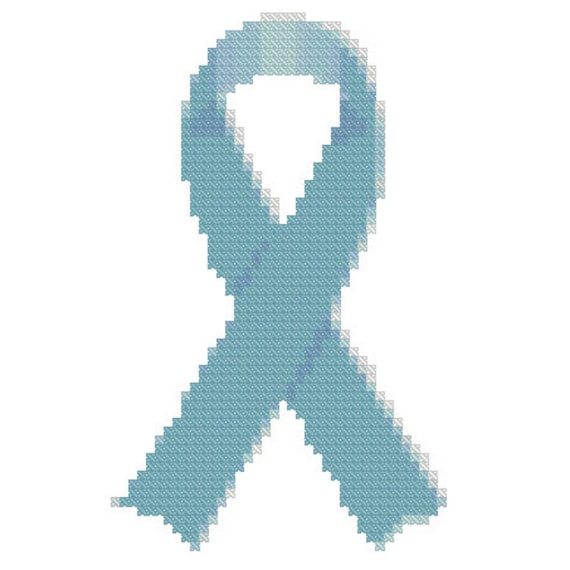The image depicts a large, bright, aqua blue awareness ribbon, rendered in a pixelated style that mimics a cross-stitch or knitting pattern. The ribbon, which seems to symbolize support for a cause, is prominently displayed on a plain white background and appears to float without being anchored to any frame or hoop. The composition of the image mirrors the textured look of embroidery, with each pixel or square meticulously forming the design. The ribbon starts from the bottom left, loops up to the top right, then back around to the top left, before crossing itself and ending at the bottom right. Notably, it features a lighter coloration at the top center, and the edges are outlined in a beige hue, adding depth and definition to the piece. The subtle shadowing where the ribbon overlaps in the center further enhances the tactile, frayed appearance, giving it a sense of dimensionality.